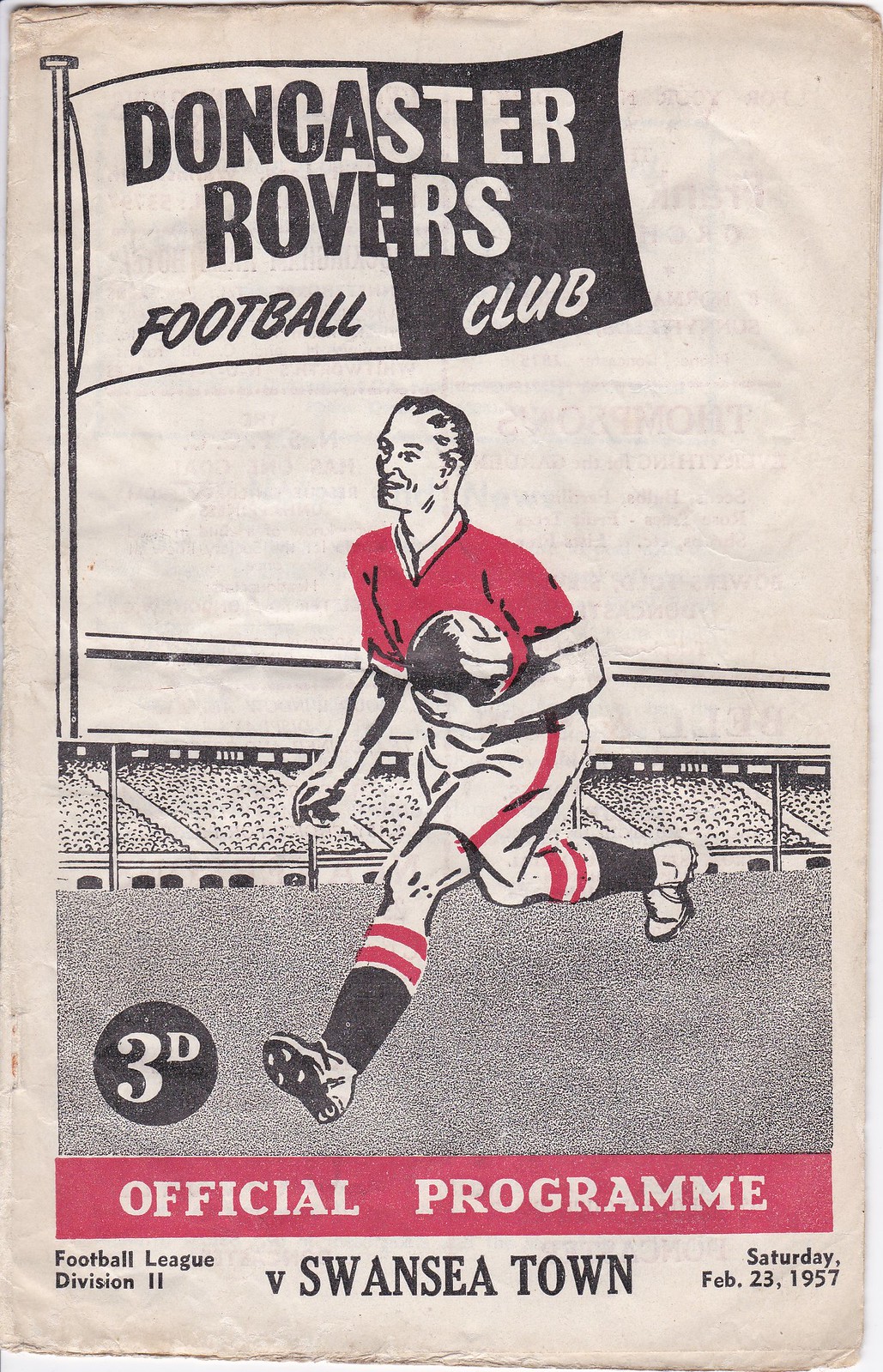This is a detailed depiction of the cover for a sports program, specifically for a soccer game, dated Saturday, February 23, 1957. The cover features a meticulously hand-drawn scene against a solid white background. In the top left corner, there is a uniquely designed flag that is vertically split into black and white halves, reading "Doncaster Rovers Football Club," with the text color inversely matching its respective background section. The flag is attached to a flagpole, which is situated next to a grandstand filled with a cheering audience.

At the center of the illustration, a dynamic figure of a man is captured mid-run, holding a soccer ball in his hands. He is dressed in a red jersey accompanied by white shorts featuring red side stripes, and his socks are adorned with black, red, and white stripes. Intriguingly, the juxtaposition of the man holding the soccer ball while running might evoke a sense of rugby rather than soccer. Additionally, positioned near his left foot is a black circle with white 3D text.

At the bottom of the cover, in bold black text, it reads: "Football League Division 2 v. Swansea Town, Saturday, February 23rd, 1957," clearly indicating the date and the competing teams for the match featured.